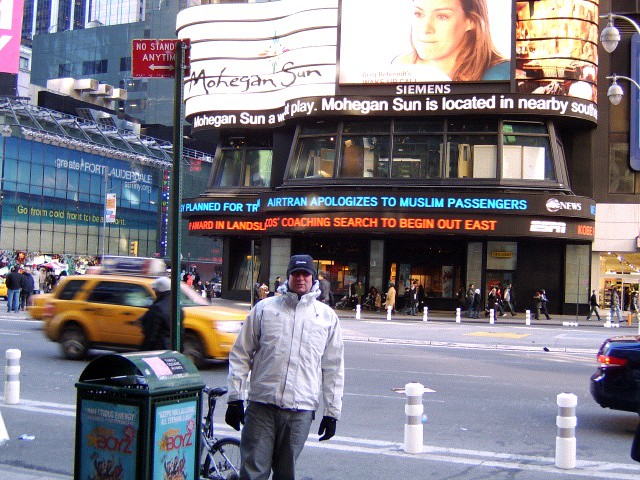The image captures a bustling city street scene centered around a man posing for a photograph. The man, dressed in a white coat, blue jeans, black gloves, and a blue cap, stands slightly to the left in the foreground, next to a trash can with an advertisement and a small bicycle parked beside it. This lively street features various vehicles, including a cab and another car with visible taillights. 

In the background, the street is lined with buildings; prominently, there's a venue named the "Mohican Sun" with billboards and horizontal message boards displaying information like news updates, including one mentioning "AirTran apologizes to Muslim passengers" and "coaching search to begin out east." Additional visible details include a metal pole installed by the street and people walking on the opposite sidewalk. Behind these pedestrians, promotional material for the company Siemens can be seen on another building. The main focus remains on the gentleman, set against this urban backdrop that highlights various elements of city life.